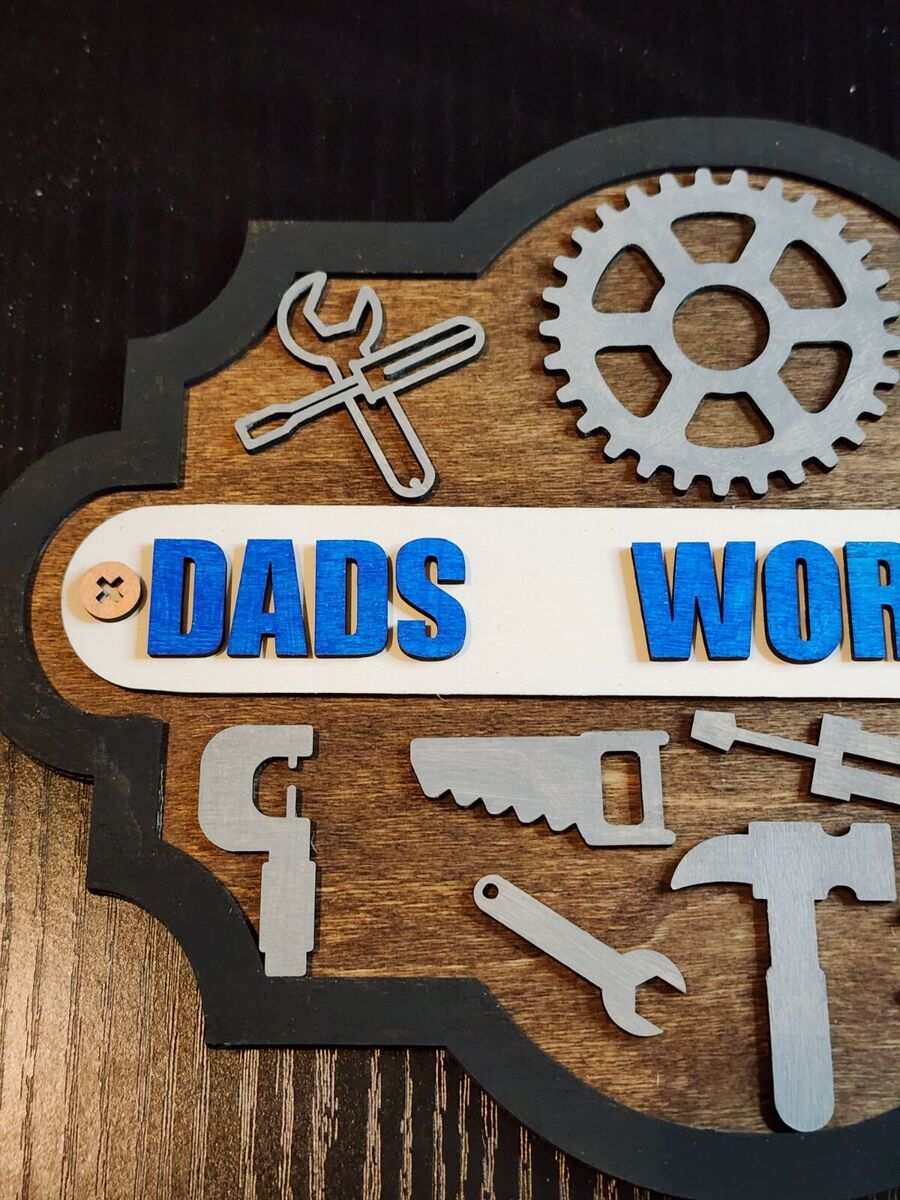The photograph depicts a meticulously crafted wooden sign, likely fashioned for a father's workshop. The sign, viewed from its partially visible left side, sits against a wooden backdrop at the bottom and a plain black backdrop at the top. It boasts a distinctive design with a thick black outline featuring both curves and straight lines. A prominent gear adorns the top of the sign, next to a crisscrossed screwdriver and wrench.

Beneath these symbols, the sign displays the partially observable text "DADS W-O-R" on a beige background, suggesting it likely reads "Dad's Workshop." Below the text, there are silver-outline representations of various tools: a saw, a wrench, a hammer, and potentially another screwdriver or micrometer, emphasizing the workshop's focus on mechanical and woodworking tasks.

The sign, bordered by a wooden frame, is intricately placed with the intention of signifying a dedicated space for the father's projects, marking it as his personal domain within the larger context, presumably a family environment.